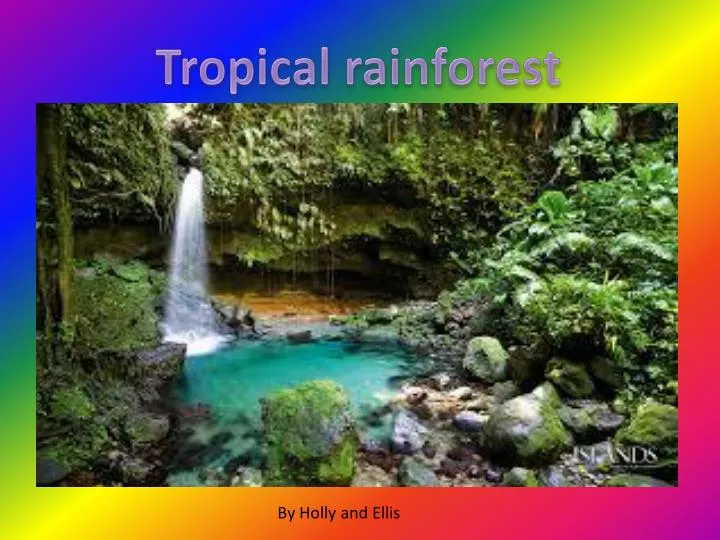The title card for what appears to be a school project showcases a vibrant and detailed depiction of a tropical rainforest. The background features a diagonal gradient with a rainbow pattern, transitioning from lilac to blue, green, yellow, red, pink, and back to purple. At the top in bold, purple font, the title reads "Tropical Rainforest." The central image depicts a lush, bright clearing abundant with diverse vegetation, including trees, flowers, bushes, and moss-covered rocks. A serene waterfall flows from a rock formation into a clear, blue pool, creating a picturesque hideaway. At the bottom of the image, the project is credited to Holly and Ellis in black text, while the word "Islands" is subtly visible in white in the bottom right-hand corner.